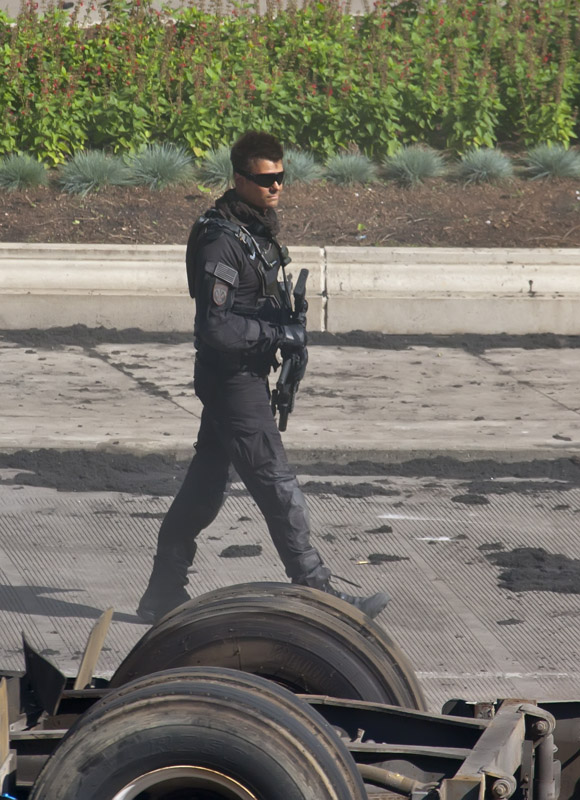The photograph depicts a SWAT officer or police officer walking along a dirty, debris-filled road. The officer, who appears to be in his mid-30s, has short dark brown hair and is dressed entirely in dark tactical gear. This includes black pants, black boots, a black vest, gloves, and dark sunglasses with black frames. He is carrying an assault rifle pointed away from the camera, and a piece of fabric can be seen around his neck. The scene is chaotic, with black dust and dirt scattered across the road, along with various grooves and lines painted on it. In the foreground, there are two large wheels, possibly related to machinery or a vehicle accident, as the metal undercarriage of what is likely a flipped car is visible. The background features a mix of greenery, including bushes with red flowers and succulents, leading up to a concrete barrier wall.